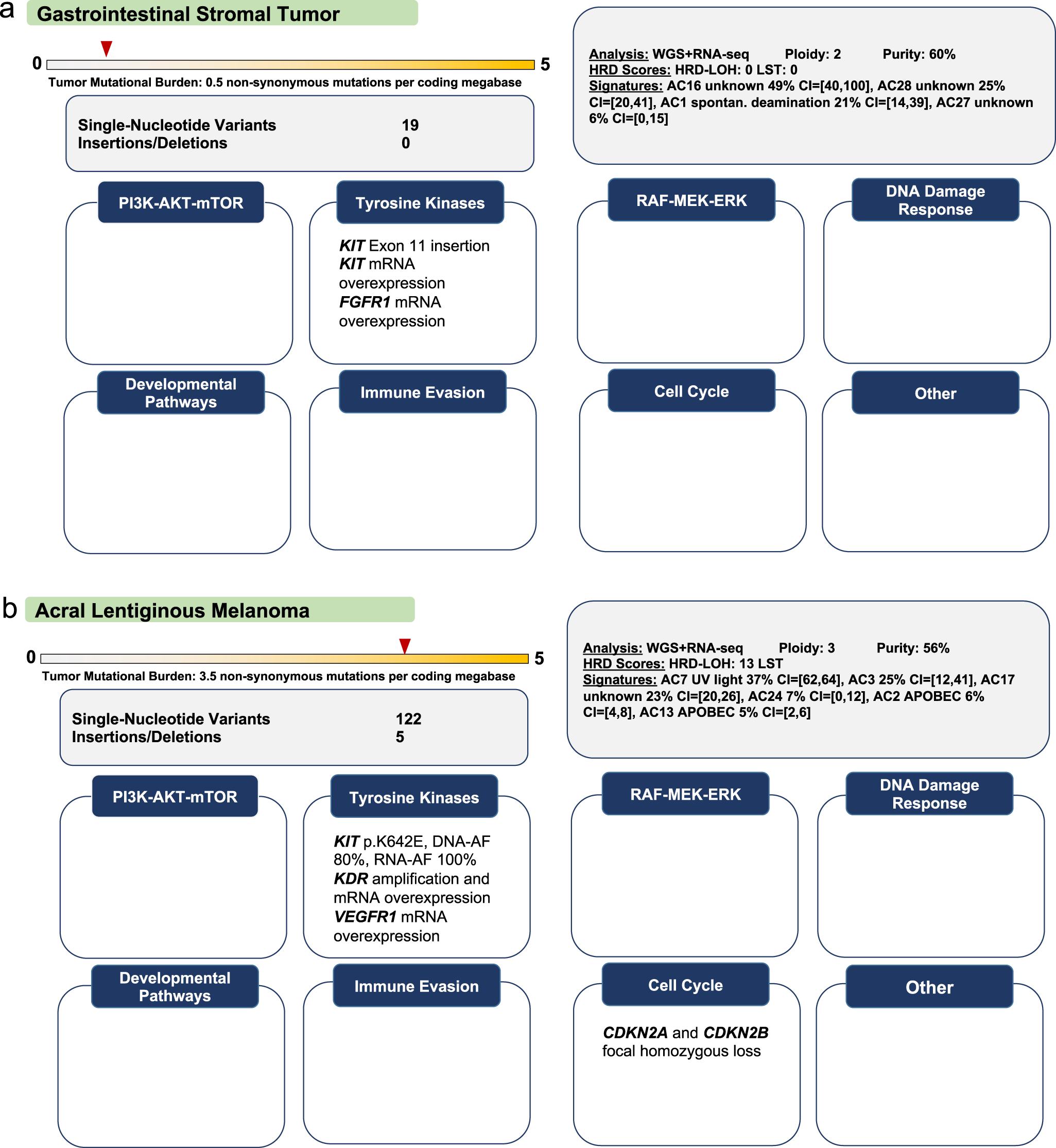The image is an instructional medical chart with multiple lines of text and two separate sections. The top section, labeled "A, Gastrointestinal Stromal Tumor," contains detailed information including tumor mutational burden, 0.5 non-synonymous mutations per coding megabase. It specifies 19 single nucleotide variants and 0 insertions/deletions, analyzed via whole-genome sequencing plus RNA sequencing. The image includes a ploidy of 2 and purity of 60%, as well as HRD scores marked as HRD LOH. The text is black against a green background, with rectangles featuring curved corners filled with grey or white, denoting different data points like "tyrosine kinases," "immune evasion," "developmental pathways," "PI3K, AKT, mTOR," and "Cell cycle, DNA damage response."

The bottom half of the chart, labeled "B, Acral Lentiginous Melanoma," mirrors the structure of the top section. It contains similar boxes with text against blue backgrounds, with details specific to acral lentiginous melanoma. The overall background of the image is white, and the titles are prominently displayed in bold letters. The consistent layout includes curvilinear-cornered rectangles, distinguishing between data-filled grey boxes and empty white boxes, all underlined by blue banners with white text.